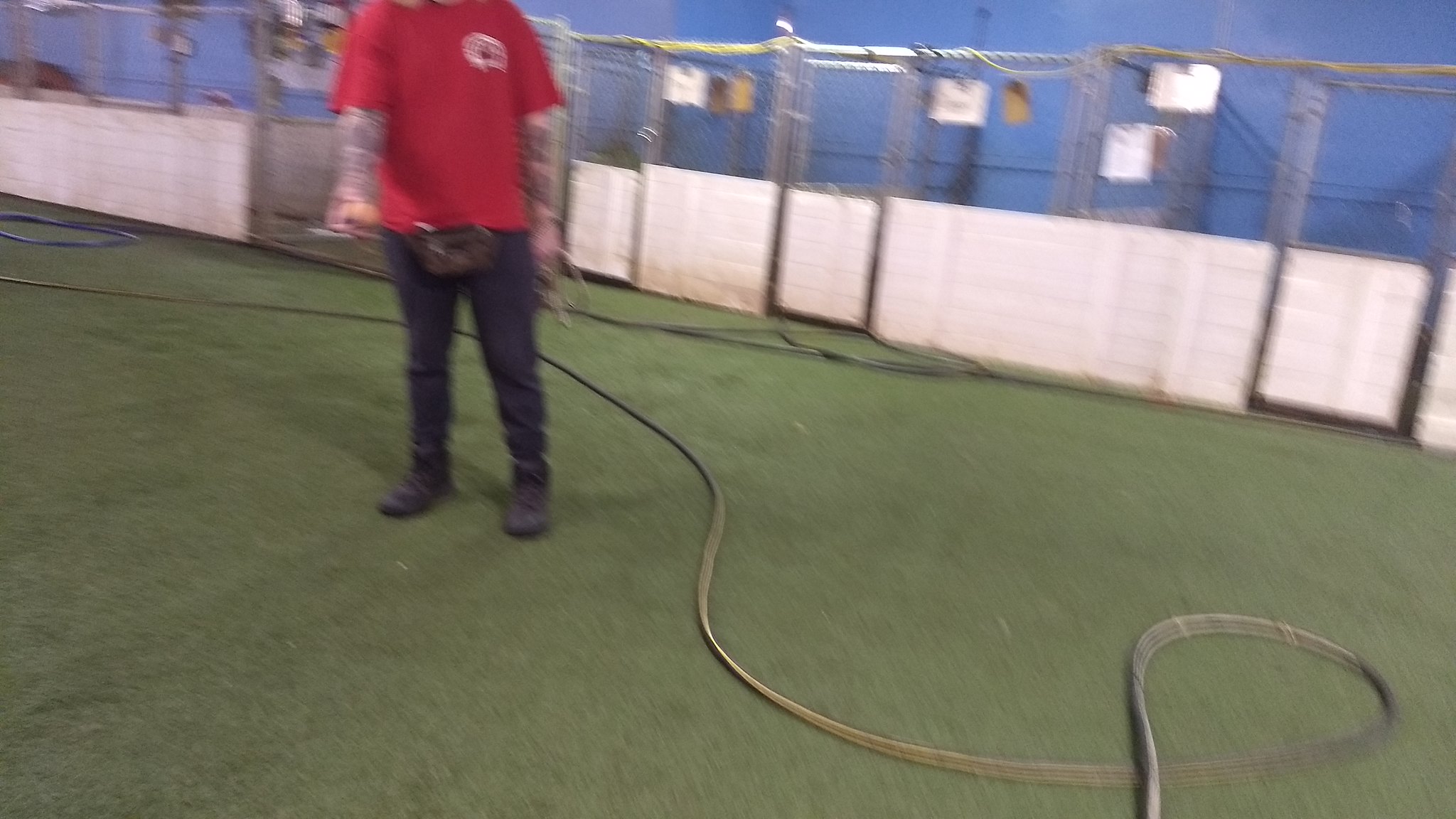In the outdoor setting of this image, a vibrant blue wall serves as the backdrop for a series of chain-link kennels, presumably housing dogs. These kennels are characterized by their cyclone fence structure, with a solid white base and small access doors. Attached to some of the kennels are signs, likely providing information about the animal occupants. Artificial grass spans the area in front of the kennels, adding a touch of greenery to the scene. A man, identifiable by his red shirt, blue jeans, fanny pack, and tattoos on both arms, is seen holding a hose. Although he is not actively spraying water, his stance indicates that he may soon begin cleaning the artificial turf. His face is not visible in the image.